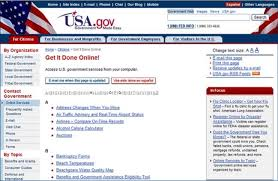This image is a highly truncated version from the USA.gov website, displaying only about 25-30% of its full content. At the top, there's a blue menu bar containing multiple options, among which one option is distinctly outlined in red. The menu options continue to extend towards the right. In the upper-left corner, there is a picture of a waving American flag in vibrant red, white, and blue, adorned with white stars. Adjacent to the flag image, the words "USA.gov" are prominently displayed, likely followed by their tagline. Above "USA," there's a comet-like emblem featuring a swoosh and a star. To the right of this, a search box is positioned, framed by some text above and below, possibly including a phone number.

Below these elements are four tabs; the leftmost tab is highlighted in red, while the remaining three tabs feature blue lettering on gray backgrounds. Beyond that, to the left side of the image, a vertical menu bar lists various options, including "My Organizations," "Something Government," and "My Reps." Centrally located, the bold text "Get It Done Online" stands out, accompanied by two buttons beneath it. Additionally, there is a directory listing with sections starting with letters "A" and "B," each accompanied by several options. To the right side, there appears to be an information section, providing further details.